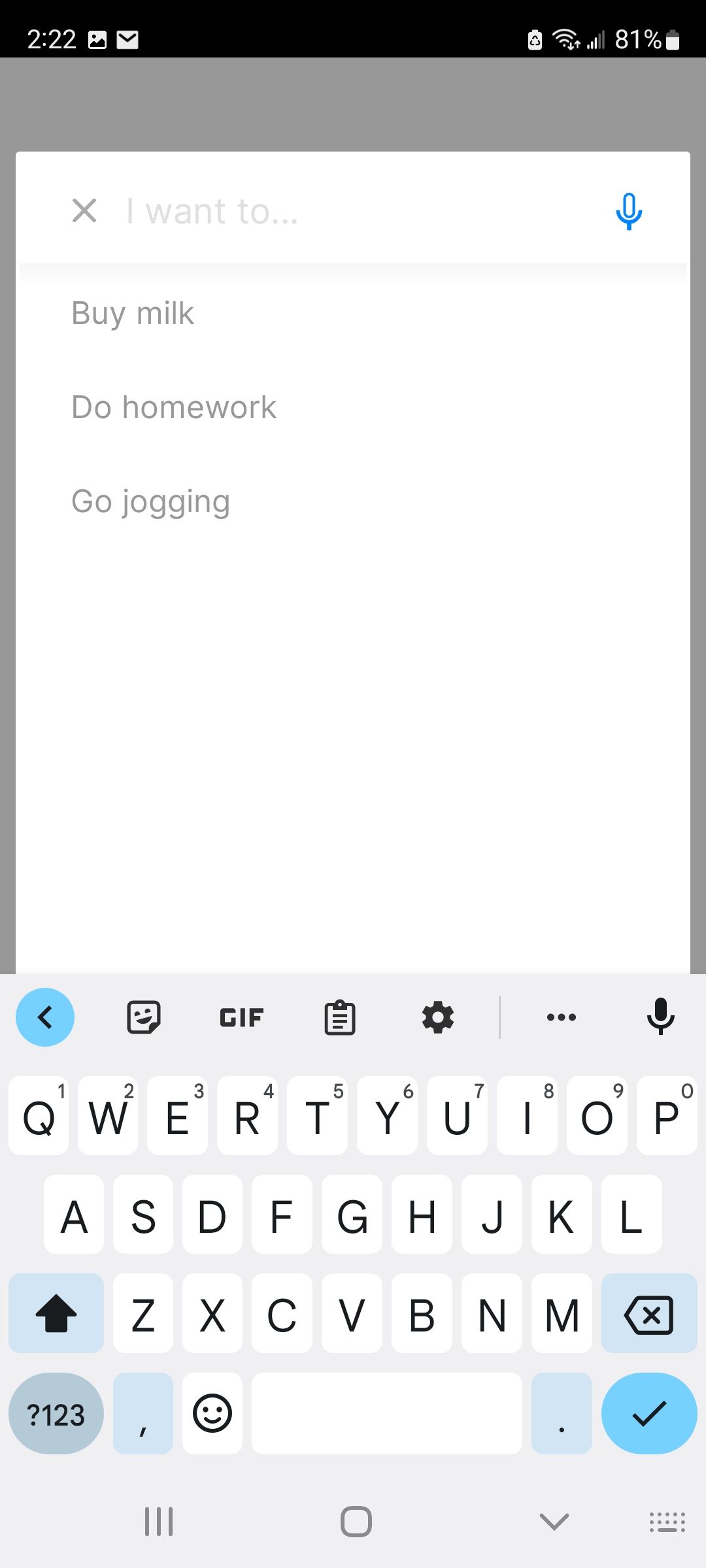The image showcases a smartphone screen with a black banner at the top of the display. The time on the phone is visible as 2:22. Positioned at the top of the screen are several app icons, including the Photos gallery tab, the Mail icon, the Wi-Fi indicator, and the battery status, which shows 81% remaining. Below these icons, a search bar is prominently displayed with the text "I want to..." entered. Next to the search bar is a blue speaker icon, indicating the option to use voice input or type in text manually.

Underneath the search bar, there is a to-do list visible with the following tasks typed out: "buy milk," "do homework," and "go jogging." Each task is neatly logged into the appropriate area, resembling a typical productivity or reminder app interface. The smartphone's keyboard is also in view at the bottom of the screen, complete with a blue circle featuring a left-pointing arrow, alongside various other icons typically found in a keyboard toolbar. The setup appears to be highly organized, aimed at helping the user manage daily tasks efficiently.